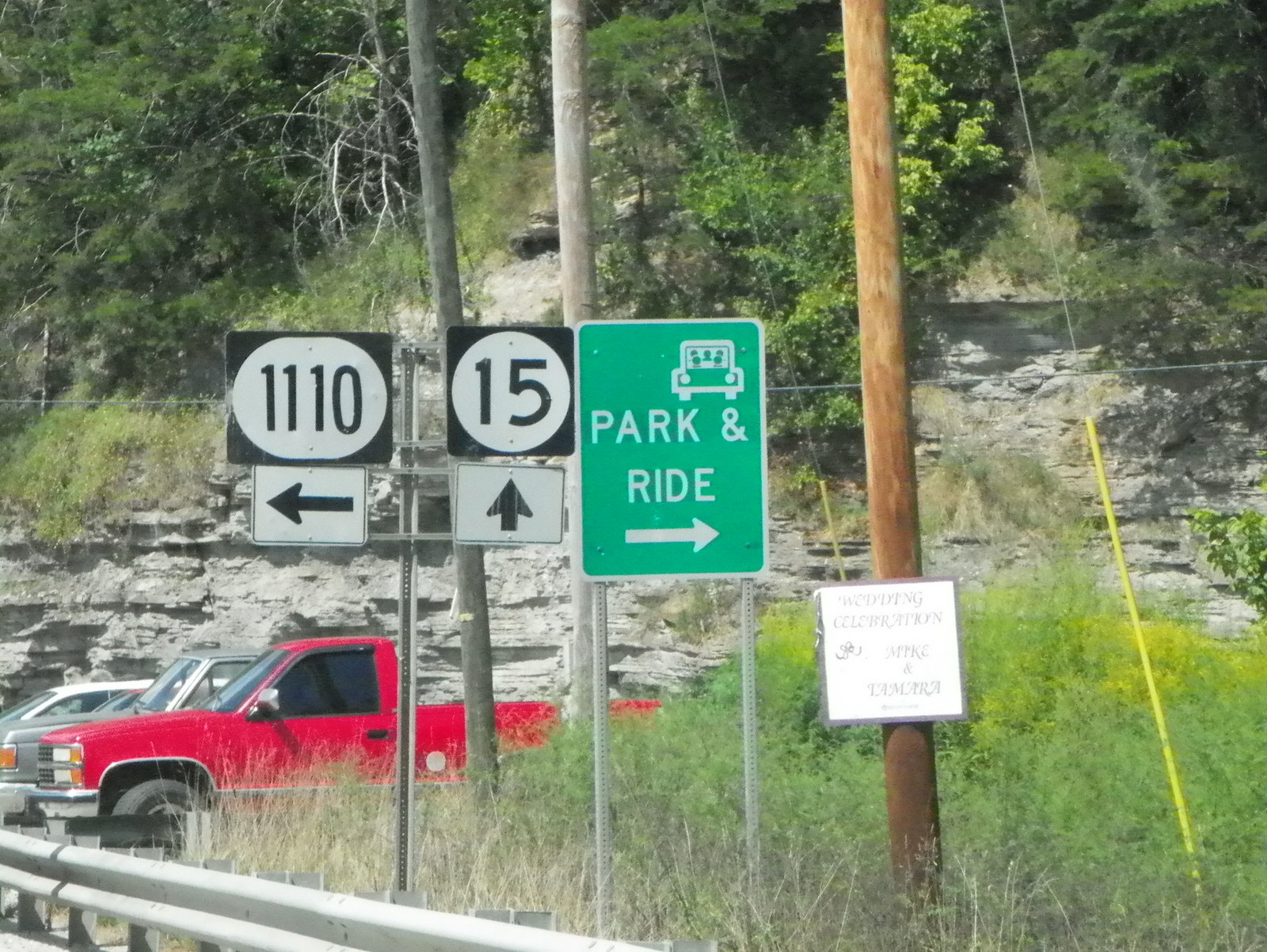On a mostly sunny day, this rectangular, landscape-oriented photograph captures an outdoor scene from a road. At the bottom of the image, a guardrail runs parallel to the road, bordered by a variety of weeds and greenery in the foreground. A wooden utility pole stands prominently, featuring a white sign that reads "Wedding of Mara." To the left of this pole, a green and white road sign, indicating a "Park and Ride" area and adorned with an arrow pointing to the right and a small automobile graphic, is mounted on double posts.

Adjacent to the park and ride sign, another single post holds two black and white highway markers. The first sign, a square with a white circle and black border, displays the number "15" and sits above a rectangular sign directing forward with an arrow. The second marker, labeled "110," is accompanied by an arrow pointing to the left.

In the background, a red truck and other vehicles are visible, contributing to the dynamic yet mundane road scene. Beyond the vehicles, trees and rocks ascend a cliff, adding a natural element to the busy roadside environment.